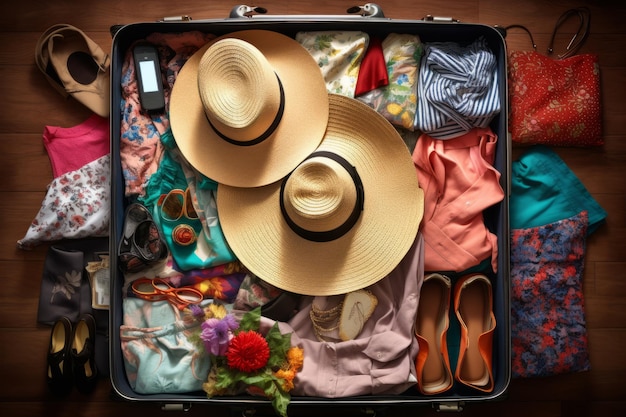This top-down photograph captures the meticulous packing of an open, square-shaped black suitcase set against a wooden floor. At the center of the suitcase, two large circular straw sun hats are carefully placed on top of an assortment of clothes, including a pink shirt and a blue and white striped shirt in the upper right. The upper left corner houses a black electronic device sitting above a pink floral garment. Nestled near the bottom, a bouquet of flowers or perhaps a brooch adds a touch of elegance. Around the suitcase, more items remain to be packed: additional clothing, a pair of black shoes in the bottom left, a couple of handbags, and sandals in the lower right. The scene exudes a sense of organized chaos, capturing the essence of preparation for an upcoming journey.